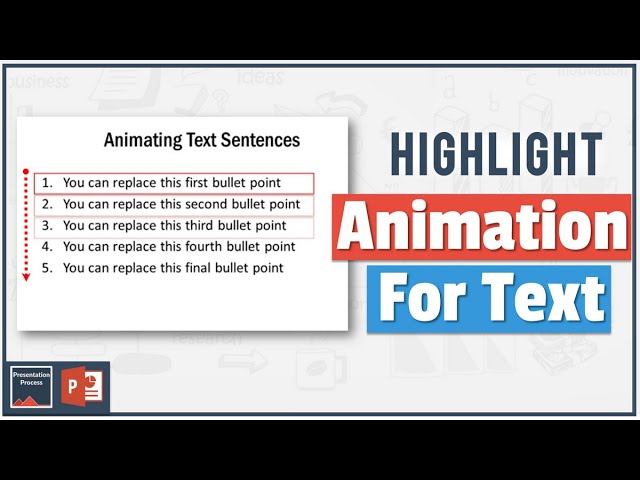The image depicts a detailed web page or instruction manual on animating text sentences, framed by thick black top and bottom borders, with additional thin blue and darker blue borders inside. The main content area has a white background. On the left side, there is a white box featuring black text, titled "Animating Text Sentences" centered at the top. This is followed by a list of numbered items: 

1. You can replace this first bullet point.
2. You can replace this second bullet point.
3. You can replace this third bullet point.
4. You can replace this fourth bullet point.
5. You can replace this final bullet point.

Adjacent to this, the phrase "Highlight Animation for Text" is prominently displayed. Below this text, a red box containing the word "Animation" in white letters is followed by a dark blue box with the words "For Text" also in white letters. In the bottom right corner, there is a dark blue square containing a white square with white text, next to an open red book displaying a large white "P" on its cover. The bottom left-hand corner of the page reads "Presentation Process."